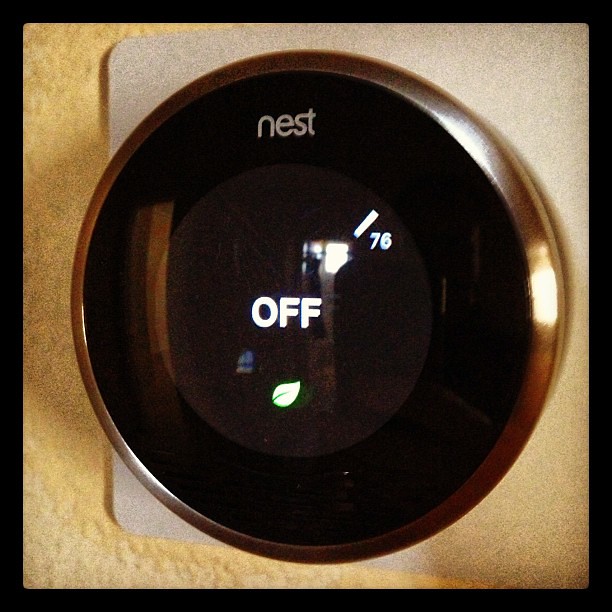A detailed photograph showcasing a Nest camera in a face-on perspective. The Nest camera, with its sleek and circular design, features a metallic edging that enhances its modern aesthetic. At the top of the camera's central display, the word 'Nest' is prominently visible, while the message 'OFF' appears in the middle of the screen, indicating its current inactive status. To the right of the 'OFF' message, slightly above, a small dash can be seen next to the temperature reading '76'. Beneath the 'OFF' message is a small green leaf icon, subtly highlighting its energy-efficient features. The camera's glossy black surface subtly reflects the surroundings, including a shadowy door and various indistinct shapes, adding depth to the image. The Nest camera is mounted on a smooth, light beige fixture, which contrasts with the light yellow, rough-textured concrete wall it is affixed to. The wall's coarse texture enhances the overall composition, providing a stark contrast to the smoother, stone-finished surface of the fixture.